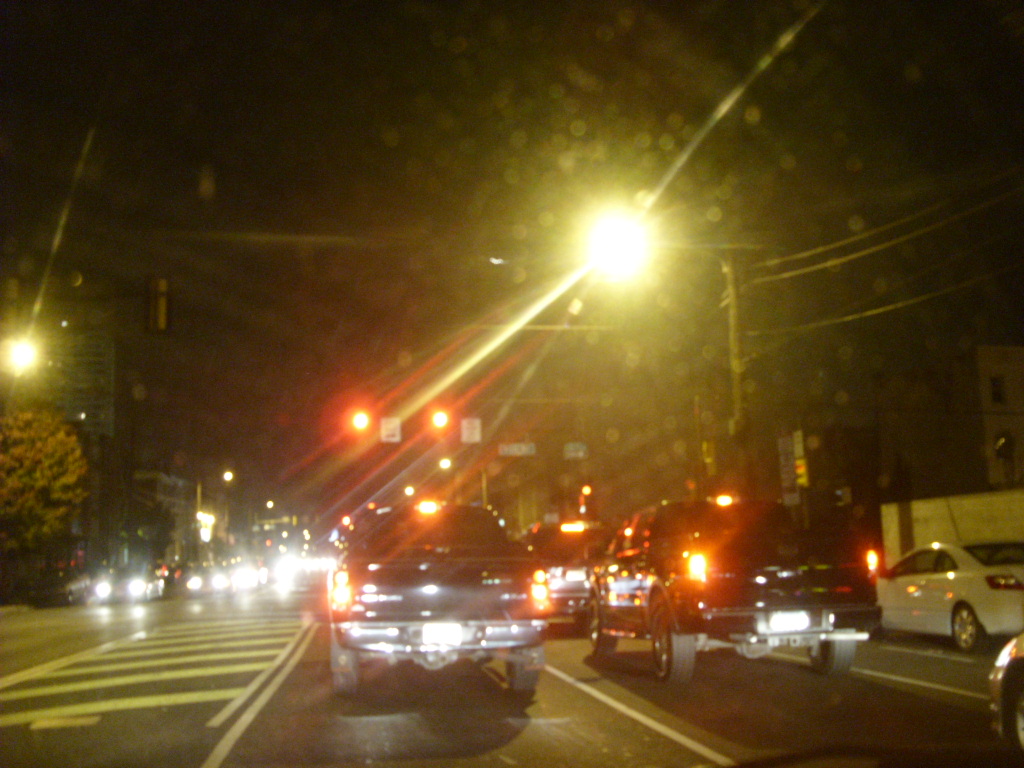The image captures a nighttime scene on a three-lane road, viewed through the windshield of a vehicle stopped at a red light. The wide photograph reveals a dark sky above, with the road illuminated by various lights. The vehicle is positioned in the left lane of traffic moving away from the camera, behind a black pickup truck, with a black SUV to the right. Headlights from oncoming traffic are visible on the other side of the intersection, which is also stopped. 

In the upper portion of the photograph, two prominent red traffic lights are visible against the black sky. A bright streetlight slightly right of center causes a starburst glare effect, casting a yellowish hue across the scene. Another streetlamp can be seen along the left side of the image. 

Additionally, the tailgate of the black pickup truck ahead reflects the headlights of the vehicle from which the photo was taken. On the right side of the photo, a white car is parked along the side of the road. The middle lane of the road, marked with yellow slanted stripes, indicates a no-go area at the red light. The overall scene is one of stillness, with all vehicles halted by the red light, and small details such as the reflections and streetlights add depth to the night-time cityscape.